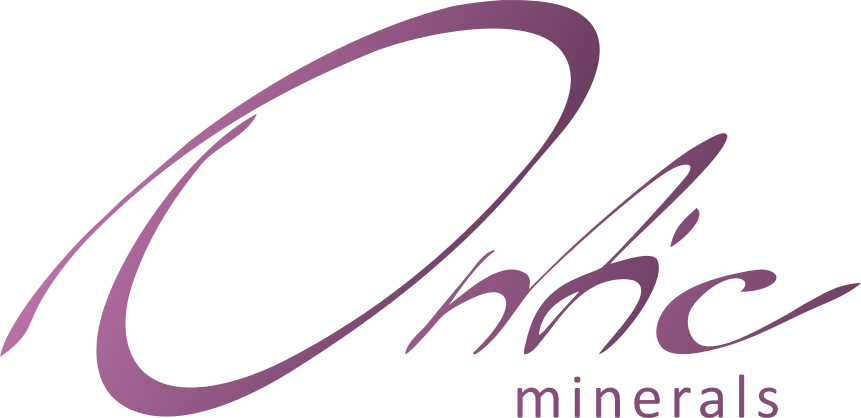The image features a bold, distinctive logo for a company, primarily colored in shades of purple against a clean, pure white background. Dominating the center of the image is a large, handwritten-style script that appears to spell out "O-N-N-C" (though the exact letters are somewhat ambiguous due to the font's flourish and possible accents). The oversized 'O' has a unique design, with a line stemming out and circling inwards beyond the initial point, giving it an artistic touch. Below this prominent script, aligned to the right-hand side, is the word "minerals" in a standard, all-lowercase font. The overall impression is of a striking and eye-catching logo meant to capture public interest in the company's offerings.